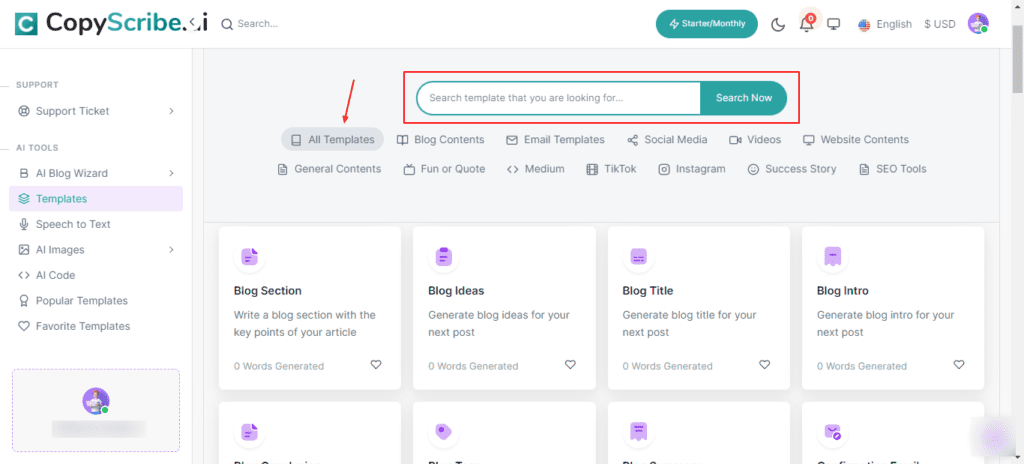A user submitted a support ticket for the Copy Scribe platform, highlighting various features and sections, including options for trials, all blogs, wizards, templates, speech-to-text functionality, images, and code. The interface includes categories such as Popular Templates, Favorite Templates, All Templates, with a prominent red arrow pointing towards it. There is also a search box demarcated by a red square, and sections labeled Starter, University, and Moon, beside components like Notifications, a Monitor, and an English US Profile Picture. General tabs include options for Bing Contents, Funner Quote, Email Template, Medium, TikTok, Social Media, Instagram, Video, Success Story, Website, Content, SEO, and Tools. Relevant Bing Sections offer suggestions for Blog Ideas, Blog Title, and Blog Intro. Additionally, users can write blog sections using the key points of their article, and generate ideas, titles, and intros for their next post. A helpful prompt invites users to post any questions they may have in the chat box for further assistance.